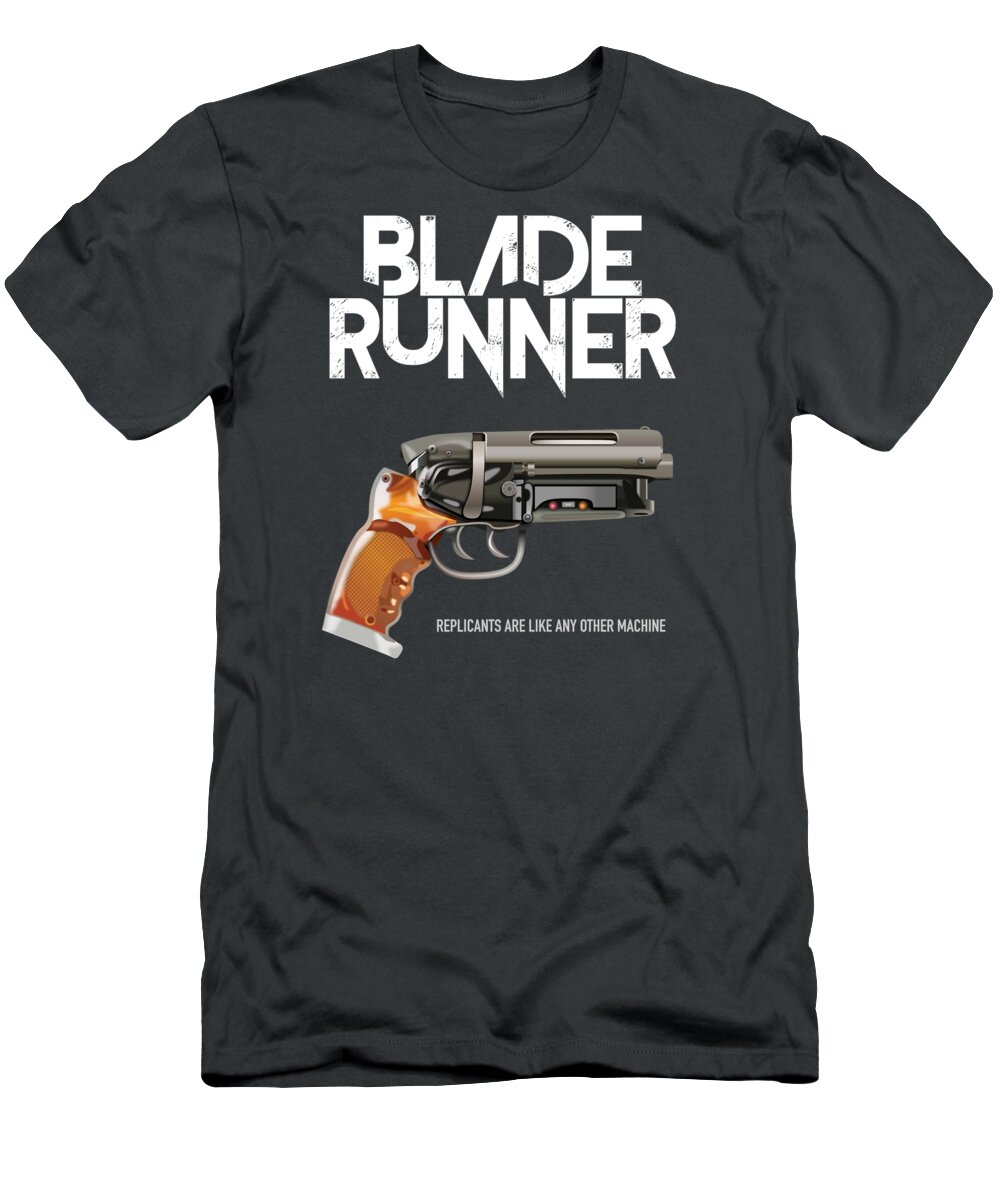The image features a black cotton T-shirt with short sleeves and a crew neck, displayed against a white background. Prominently positioned at the top center in bold white letters, "Blade Runner" is written across two rows. Directly below, there is a detailed profile of a handgun. The gun features a dark gray, thick barrel with a distinctive red and orange dot, a silver bottom, and a brown handle, and it notably has two triggers. Beneath the gun, in smaller all-caps white text, the phrase "Replicants are like any other machine" is printed. The T-shirt appears slightly wrinkled around the sleeves and bottom, but the image and text design are smooth and well-ironed. The overall setting is well-lit, enhancing the clarity and details of the T-shirt.